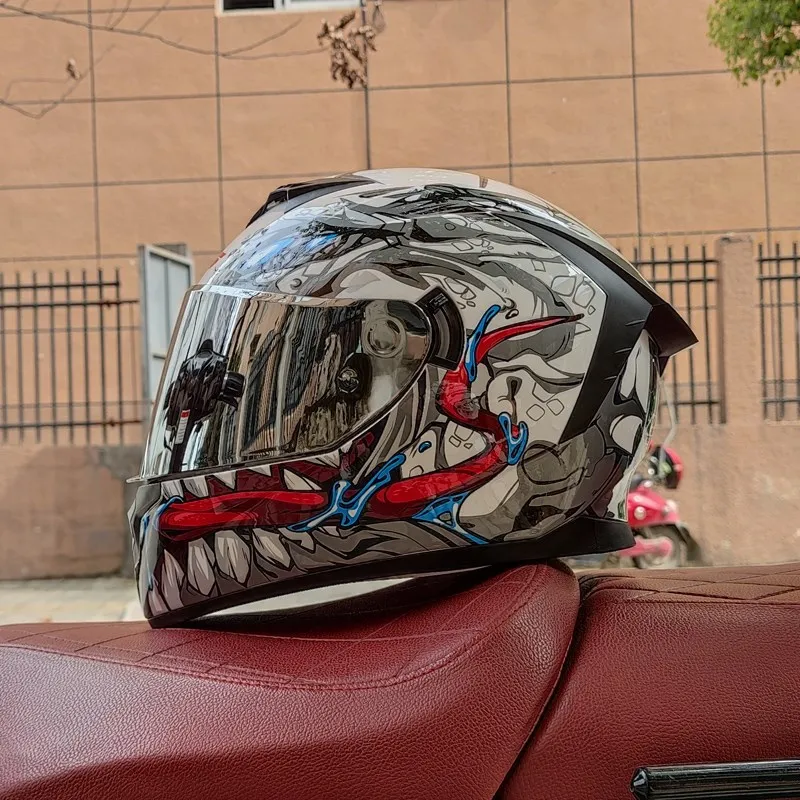The photograph features an up-close shot of a stylish motorcycle helmet resting on a deep maroon leather motorcycle seat, with a partially visible black section of the bike. The helmet, predominantly black with elaborate Marvel comic-type illustrations in striking red, blue, and white, stands as the focal point. It boasts a gleaming, highly reflective visor that mirrors parts of the surrounding environment. The lower part of the helmet features monster-like teeth and a long tongue drawing, extending to the side, with scales adorning the white areas, creating an intriguing lizard or monster motif. In the background, a dark beige building with large stone bricks and gray lines, enclosed by a metal fence atop a concrete base, adds depth to the scene. There’s also a glimpse of another motorcycle parked next to the building, further enhancing the outdoor setting. A few leaves from a nearby tree can be seen descending, complementing the urban ambiance.